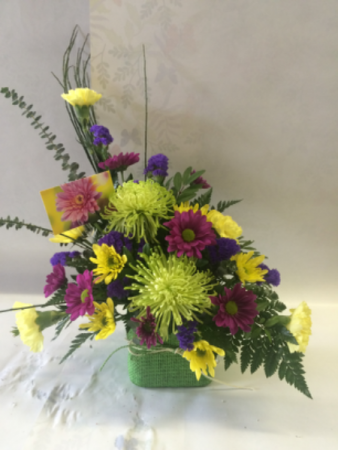This painting captures a detailed flower arrangement in a square green basket vase adorned with a twine bow. The bouquet features bright yellow, mauve, and purple flowers, complemented by green stems and decorative fern-like foliage. It sits on a white cloth, possibly a table cover, against a predominantly white backdrop with a subtle leaf design, suggesting either a reflection or wallpaper. The painting is vertically rectangular, perfect for hanging in a home. Additionally, a small card, likely indicating the sender, is nestled among the flowers, emphasizing the personal touch of this vibrant display, which could be for an occasion like a birthday, hospital visit, or graduation celebration.